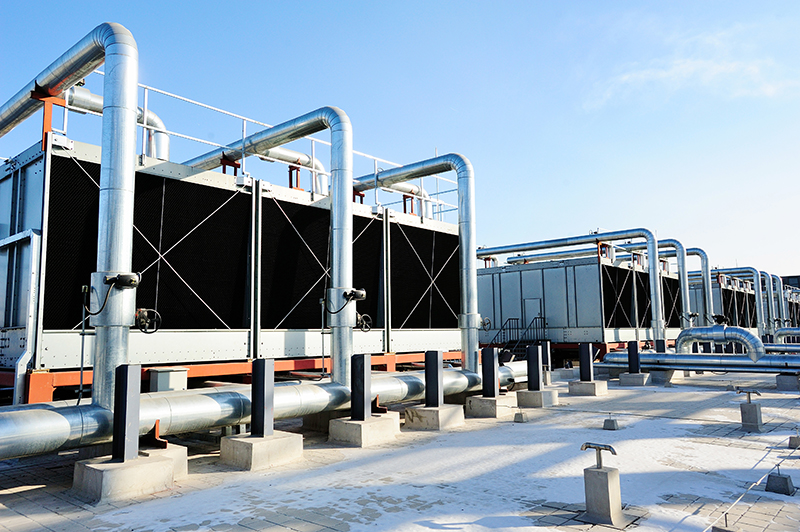The photograph captures a daytime scene on the rooftop of a presumably tall and secluded building, featuring a row of industrial air and water-cooled chillers for an HVAC system. These chillers, which appear mostly silver with black panels, are mounted on orange risers and connected by numerous sturdy metal pipes. The rooftop, paved with cement blocks, has a light dusting of snow, enhancing its clean and well-maintained appearance. The sky is bright blue with a few wispy clouds scattered sparsely, contributing to the clear and crisp atmosphere. The angle of the image suggests a diagonal view, with the chillers progressing further into the distance towards the right side of the frame.